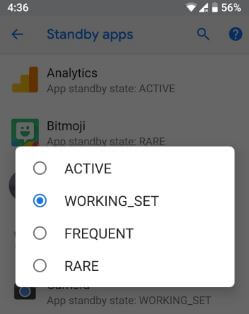The image shows a smartphone screen with a gray overlay indicating it is in a settings menu, specifically focusing on "App Standby State." The battery is at 56% and there is a strong Wi-Fi connection. The main display features a white pop-up window, which is overlaying the standby apps section. The pop-up window includes selectable options, each preceded by circles: 

- "Active" 
- "Working_Set" (which is selected and highlighted in blue) 
- "Frequent" 
- "Rare"

Beneath this pop-up, partially visible, are app-specific standby states presented in a list format:

- "Analytics app: Standby state: Active"
- "Bitmoji app: Standby state: Rare"

The bottom of the pop-up reiterates "App Standby State: Working_Set." 

The screen features various colors, including blue, orange, yellow, green, white, black, and gray, which likely represent different UI elements and statuses. This image is clearly from a smartphone settings menu, specifically showcasing the management of app standby states.